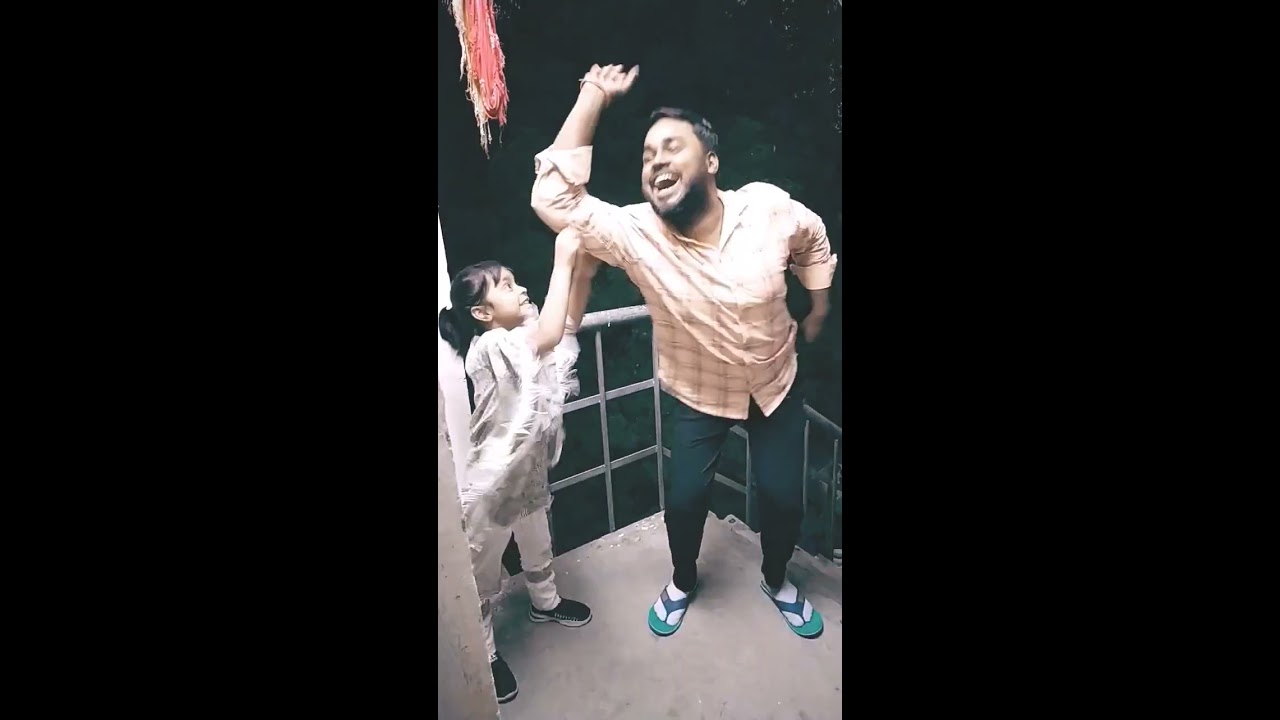In this full-color, horizontally rectangular photograph, two individuals, a man and a young girl, are captured standing at the top of a staircase with white railings. The background is predominantly black, flanked by tall, vertical black panels creating a triptych effect. The scene appears to be outdoors at night, illuminated by a spotlight that emphasizes the subjects. 

The man, who has a medium to dark skin tone and black hair neatly trimmed, is depicted leaning back with his eyes closed and mouth wide open in a joyful laugh. He sports a trimmed beard and is dressed in flip flops, possibly white socks, blue or dark pants, and a long-sleeved shirt in an off-white or salmon hue, with the sleeves rolled up to his shoulders. His right arm is raised high in the air, and the little girl, around seven years old, is holding onto it with both hands while grinning widely. 

The girl is dressed in white pants and socks, black shoes, and a light-colored shirt adorned with a feather boa scarf across her chest. Her dark hair is tied back into a ponytail. Above them, a red and yellow feathery cloth descends from the ceiling, contributing a whimsical element to the scene. The image captures a moment of shared exuberance between the man and the girl against the contrasting dark background.